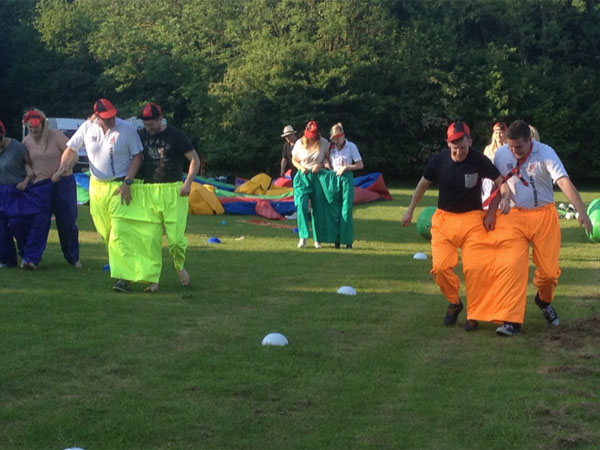The photo captures a vibrant, outdoor summer event set in a lush green park. Four to five groups of adults are engaged in a spirited three-legged race, navigating an obstacle course on a well-maintained grass lawn. Each pair wears a comical oversized pair of three-legged pants, which are two pants sewn together with a shared central leg, requiring teamwork and coordination to move. The visible participants sport a variety of brightly colored pants—orange, green, yellow, and dark blue—adding a festive touch to the scene. They are also wearing amusing black and red baseball caps. The background features thick, green-leaved trees, with the sunlight casting a serene glow on the leaves in the middle. Additionally, a deflated inflatable structure is faintly visible, adding to the lively atmosphere of this team-building event.